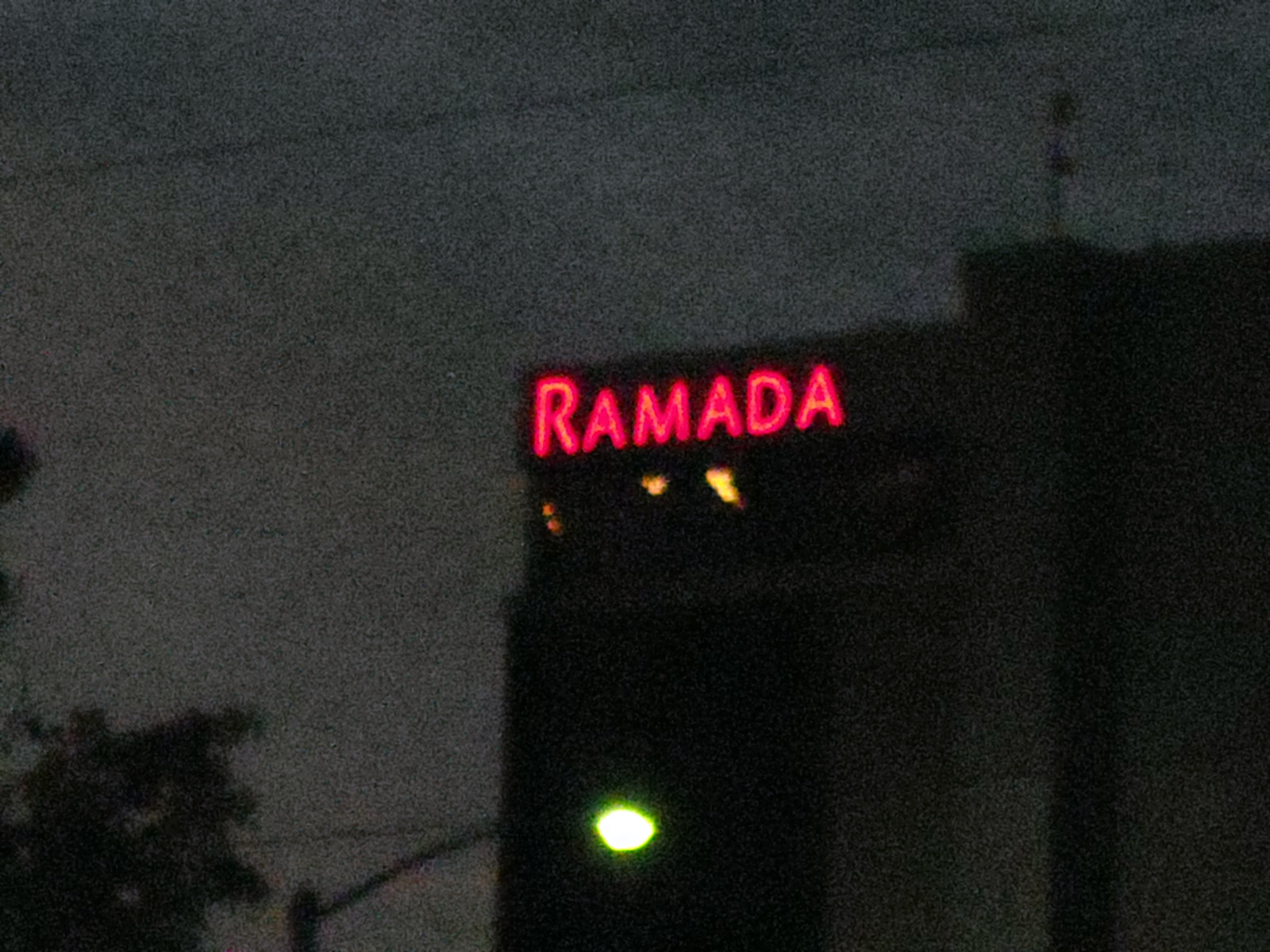This grainy, low-quality nighttime photograph depicts a Ramada hotel. The dark, black sky enhances the gritty appearance of the image, while a greenish-yellow street lamp illuminates the foreground, casting light on the scene. The Ramada hotel building is positioned from the left, extending vertically and horizontally, covering half of the image. The iconic Ramada sign, in internally illuminated red capital letters, dominates the upper left-hand corner of the building, with the letter 'R' being conspicuously taller than the rest. Below the sign, three yellowish lights are visible, possibly illuminating the letters 'R', 'A', and 'M'. The hotel’s top features various objects, including antennas and cables, which stand out against the dark sky. The lower left corner of the image shows the silhouette of tree leaves and branches, adding to the overall dark and murky atmosphere. No other lights are visible on the building, leading to the assumption that any internal lights are either turned off or non-functional.